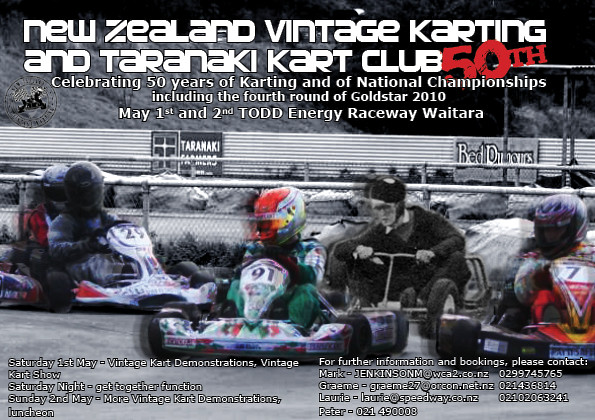The flyer advertises the New Zealand Vintage Karting and Taranaki Kart Club's 50th anniversary event, celebrating half a century of karting and national championships, including the fourth round of Gold Star 2010. The event will take place on May 1st and 2nd at Todd Energy Raceway, Waitara. The design features a central photograph of four to five go-kart racers, with the riders in color and the background in black and white, providing a vivid contrast. Some of the go-karts display bright trims in green, red, and blue, against the otherwise monochromatic backdrop. 

The text at the top of the flyer reads: "New Zealand Vintage Karting and Taranaki Kart Club, 50th," in a mix of white and red text. Below it, the flyer details the celebration: "Celebrating 50 years of karting and national championships, including the fourth round of Gold Star 2010, May 1st and 2nd, Todd Energy Raceway, Waitara."

Further information is provided at the bottom, detailing the schedule: "Saturday, May 1st, Vintage Kart Demonstrations, Vintage Kart Show, and Saturday Night Get Together Function. Sunday, May 2nd, More Vintage Kart Demonstrations and Luncheon." Contact details for further information and bookings are listed on the right side of the flyer, including names such as Mark Jenkinson and others, along with their email addresses and phone numbers.

The photo composition includes go-karts on a track with fencing visible, and there's a blend of modern and vintage elements to showcase the 50-year history.